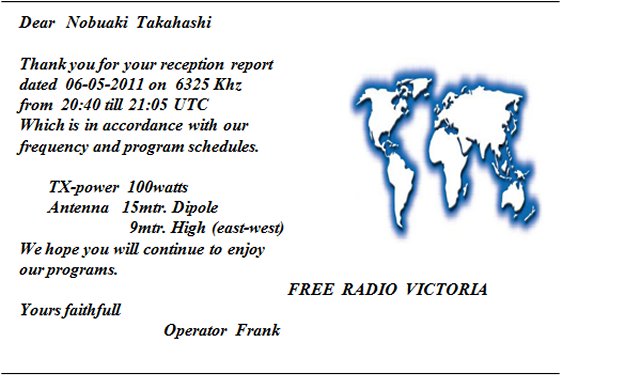This image features a detailed receipt card prominently displaying black text on a white background, delineated by thin black lines at the top and bottom. To the top left, in italic script, it reads: "Dear Nobuaki Takahashi, thank you for your reception report dated 06-05-2011 on 6325 kHz from 2040 till 2105 UTC, which is in accordance with our frequency and program schedules. TX power: 100 watts, Antenna: 15-meter dipole, 9 meters high, east-west. We hope you will continue to enjoy our programs. Yours faithfully, Operator Frank."

Adjacent to this text, in the top right corner, there is an illustrated map of the world. The continents—North America, South America, Europe, Asia, Africa, and Australia—are depicted in white with black outlines, surrounded by a blue glowing effect. Beneath the map, in all capital letters and still in italics, the card states: "FREE RADIO VICTORIA."